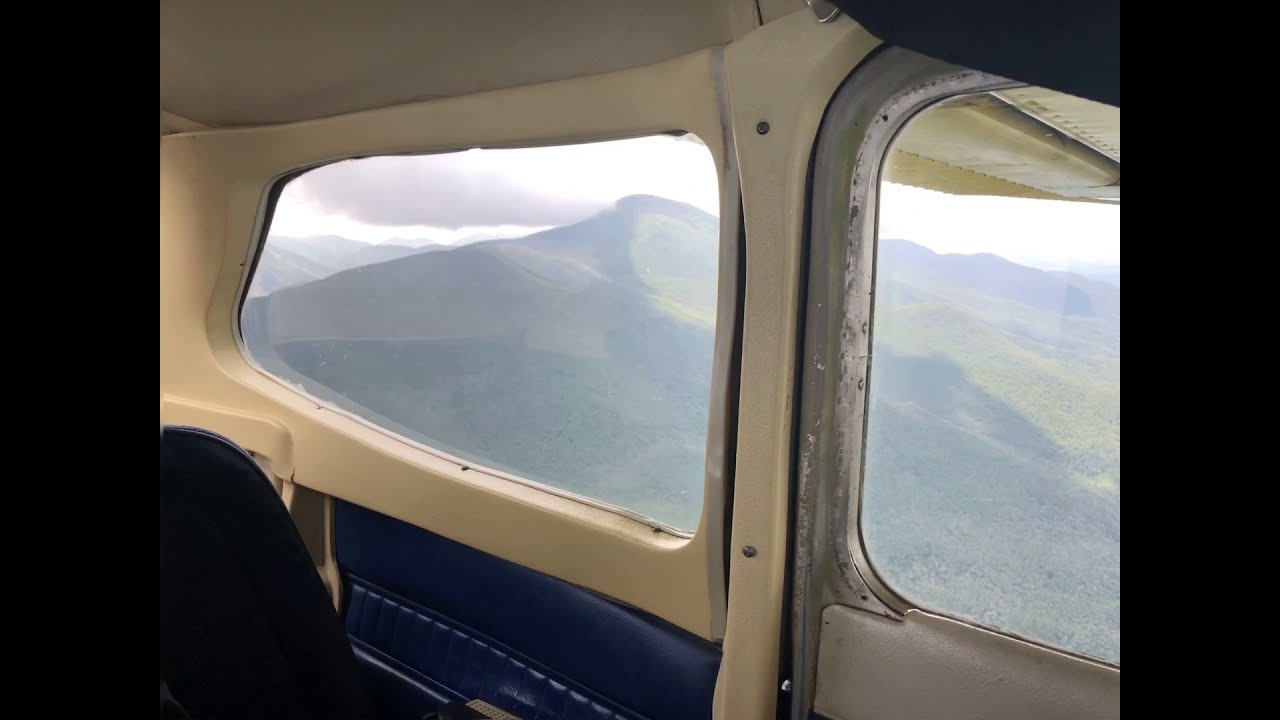The image depicts the interior of a small Cessna-type propeller plane. The interior is predominantly white with some blue upholstery on the arm panels next to the seat. To the right, there is a worn metal door featuring a silver finish and a rounded square window. Behind it, a more rectangular window is visible. The cabin is cozy, reflecting the compact nature of the aircraft. In the lower left corner, part of a black seat can be seen. 

Through the windows, a scenic view of lush green mountains unfolds, covered in vegetation and basking in natural sunlight with noticeable glare. White clouds hover above the mountain peaks, and a wing of the plane is partly visible, suggesting the aircraft is in flight and possibly on a sightseeing journey. The sky outside is a patchy blue-gray, adding to the serene atmosphere. The array of colors both inside and outside the plane includes shades of white, blue, green, tan, gray, black, and silver. 

Overall, the image captures a tranquil aerial view juxtaposed against the slightly worn and intimate interior of the small aircraft, providing a sense of both adventure and aged charm.